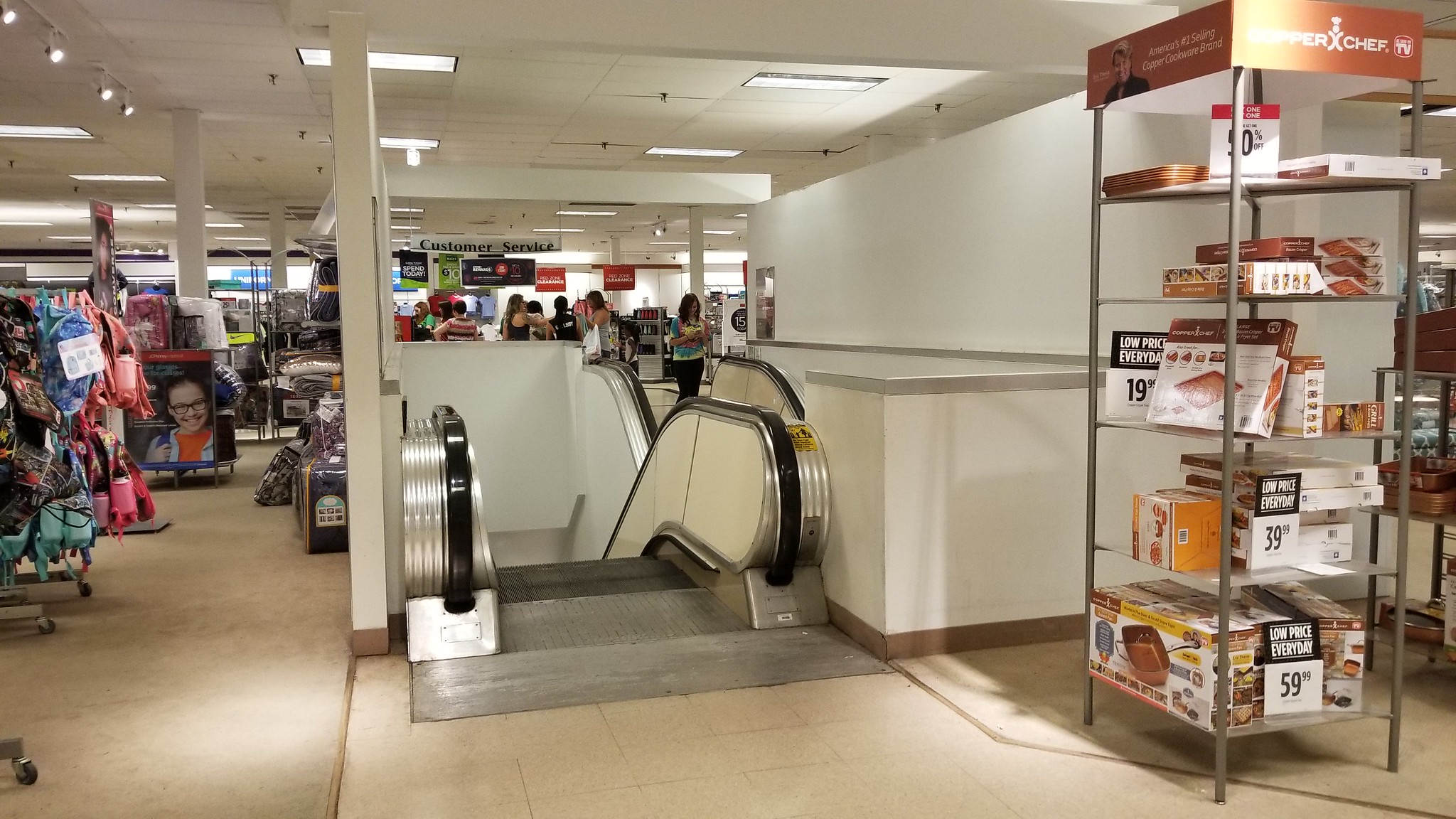The image captures a bustling department store centered around a set of escalators. The main focus is on an escalator with black handrails descending to a lower level, while a second escalator mirrors it in the background, ascending. The flooring transitions from a light brownish tile to a matching carpet. On the right side of the image stands a prominent metal shelf with five tiers, topped by a bronze sign that reads "Snapper Chef." Each shelf displays boxed products priced at $59.99, marked with tags that read "low price every day" in black text against a white background. The left side features additional racks showcasing a variety of merchandise, including pillows, backpacks, and assorted clothing. Shoppers move throughout the background beyond the escalators, and a faint white sign hanging from the ceiling indicates the customer service area with a lineup of about ten women. The store's interior is brightly lit with recessed lights, set against clean white walls and an off-white ceiling. Various sale signs are strategically hung, adding to the lively commercial atmosphere.